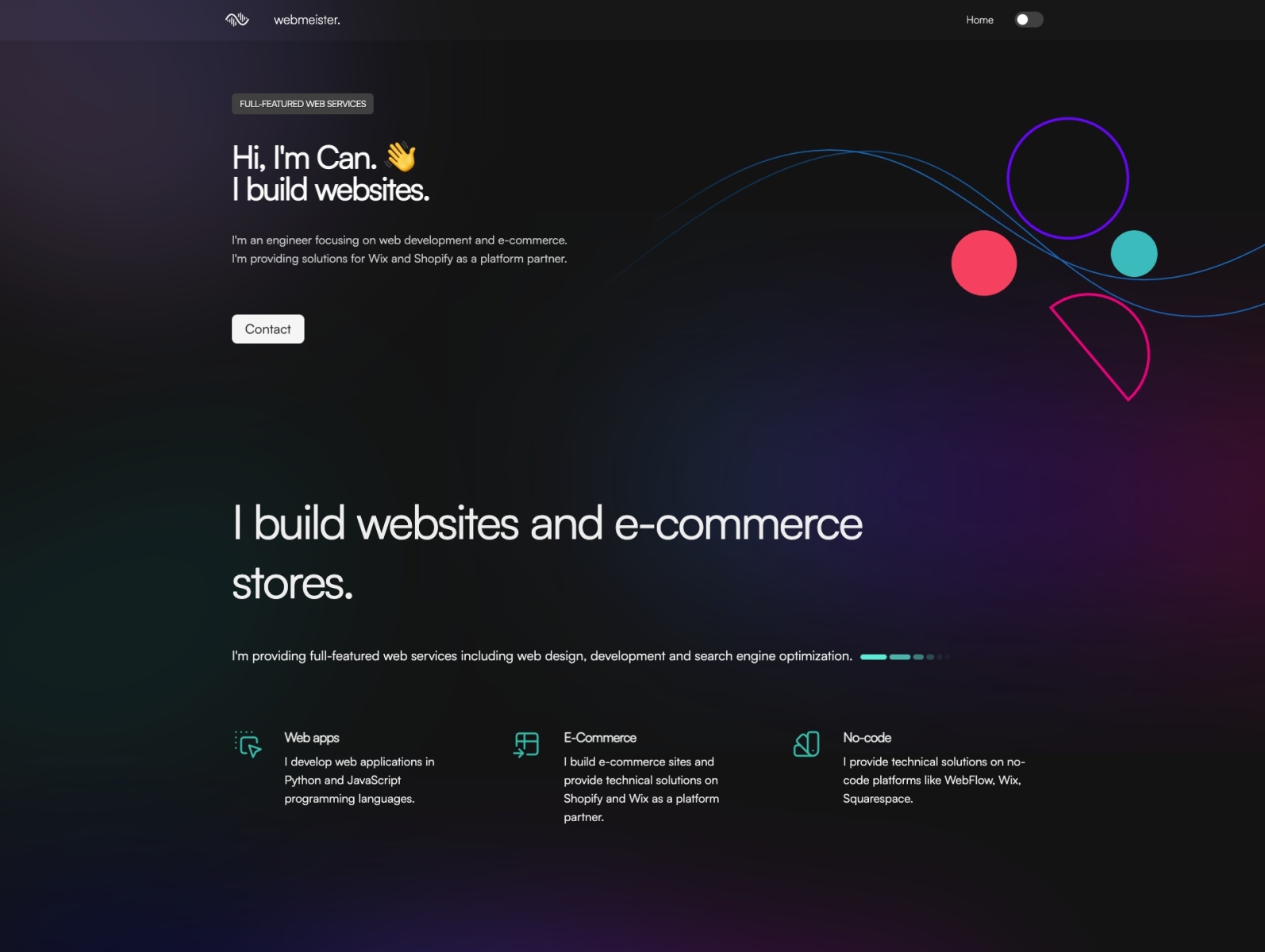This image appears to be a screenshot from the website "Web Meister". The background is a gradient blend of dark blue, reddish-purple, and dark purple hues. 

At the top section of the image, a header bar spans across the image. This bar features a white logo on the left side, followed by the text "Web Meister" also in white. On the far right, there is a home button adjacent to a white switch that is currently in the "off" position, likely indicating a control for light or dark mode on the site.

Beneath the header, on the left side, there is a section titled "Full Featured Web Services". The text reads: "Hi, I'm Ken" followed by a waving emoji. It continues to describe Ken as an engineer specializing in web development and e-commerce, offering solutions as a platform partner for Wix and Shopify. Below this text is a white "Contact" button.

On the right side of the image, there are several graphic elements, including a red half-circle, a full red circle, a smaller teal circle, and a large outlined purple circle with a black center.

Further down, additional information is provided about e-commerce and web building procedures. The layout and colors create a visually engaging introduction to the services offered by Ken on the Web Meister website.